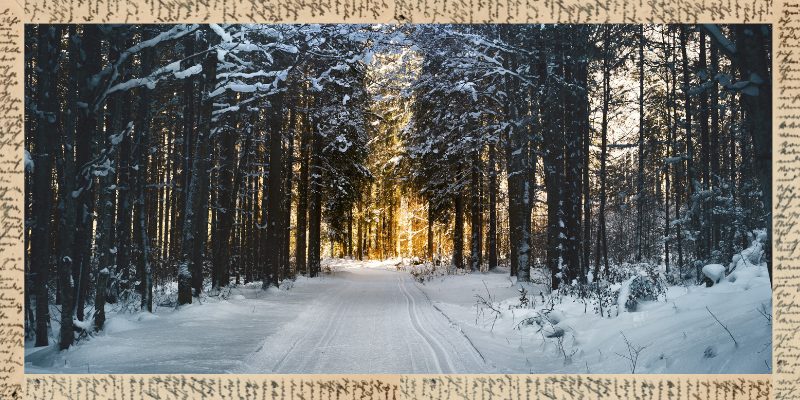This is a horizontal color photograph capturing a serene winter scene within an old-growth pine forest, adorned with an artistic border resembling brown paper covered in unreadable cursive script. The densely populated trees, their dark, nearly black trunks contrasting sharply with the blanket of snow, create an almost monochromatic palette of white and dark hues, emphasizing the stark beauty of winter. A snow-covered road bifurcates the forest, its wavy, streaked tracks suggesting recent plowing or vehicle passage. The branches of the towering, slender pines are heavily laden with snow, adding to the somber beauty of the landscape. In the background, the dense canopy gives way to a brighter, golden light, hinting at a clearing or the promise of the day's end. The handwritten script surrounding the image adds a touch of historical or artistic intrigue, making the entire composition feel both timeless and contemplative.